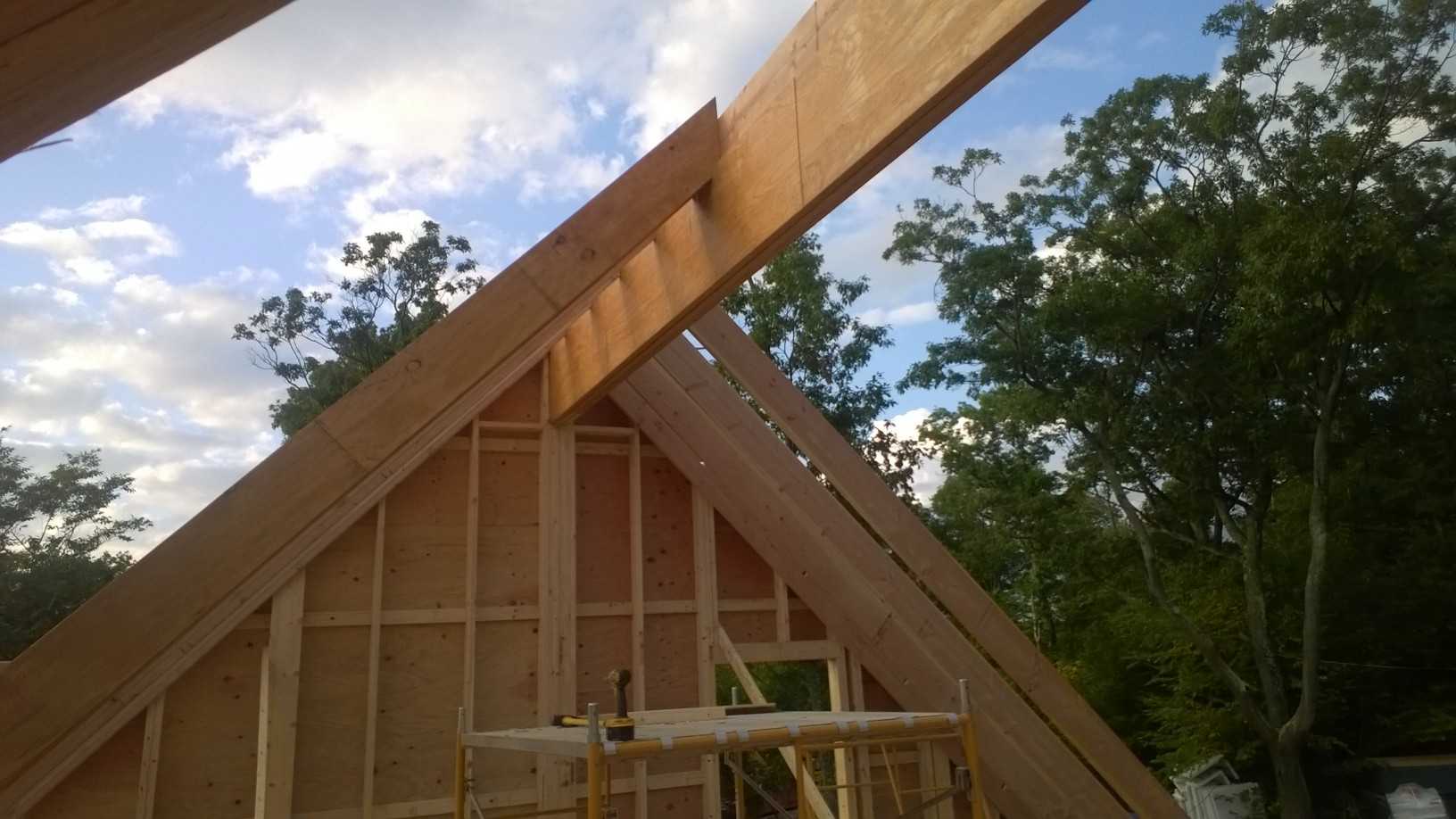The image depicts an A-frame house under construction, showcasing a central truss beam running lengthwise along the peak of the roof. Smaller angled beams connect to this main beam, descending towards the outer edges. The back wall features a rectangular pattern made from 2x4s to ensure structural support, evenly spaced about 2 feet apart. Midway up the wall, a horizontal beam provides additional stability.

In the center of the construction site, there is a makeshift wooden table cluttered with work supplies, prominently including a yellow drill and a yellow hammer. The background of the scene is dominated by tall, green coniferous trees under a blue sky with large, white clouds. Notably, there are no people visible in the photo, though the presence of scaffolding and tools suggests active construction work. Near the right side, some white objects are partially visible, but their exact nature remains unclear. 

The ongoing project reflects early construction stages with its exposed framing and vibrant, pine-colored wood, emphasizing the skeletal structure of this emerging A-frame house.